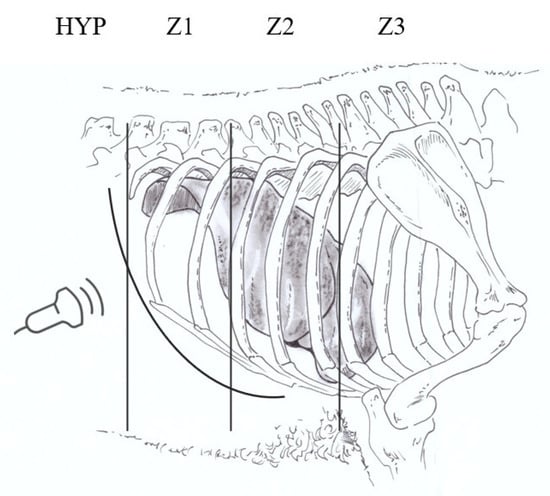The image is a detailed black-and-white sketch featuring the skeletal structure of an animal, most likely a dinosaur or a large mammal. The central focus of the drawing is the rib cage and part of the spine, with bones of the front leg also visible on the right side. The background is stark white, making the black outline and the few colored elements stand out prominently. At the top, the labels "HYP, Z1, Z2, and Z3" are written in capital letters, likely indicating different sections of the spine or rib cage.

Above the rib cage, three vertical lines are marked, perhaps as part of some measurement or annotation. On the left side, there's a symbol resembling a bell with two lines in front of it and a string attached to its end, which might be interpreted differently as an ultrasound icon or even a thumbtack or needle. Inside the rib cage, there’s a reddish-colored area which could signify an internal organ or tissue.

The drawing is quite detailed, even showing the leg bones and additional ribbing towards the top of the image. There’s also some grass sketched at the bottom, adding to the naturalistic elements of the sketch. The entire composition is meticulous, with the only colored part being the red detail inside the ribs, contrasting against the otherwise grayscale and white palette.